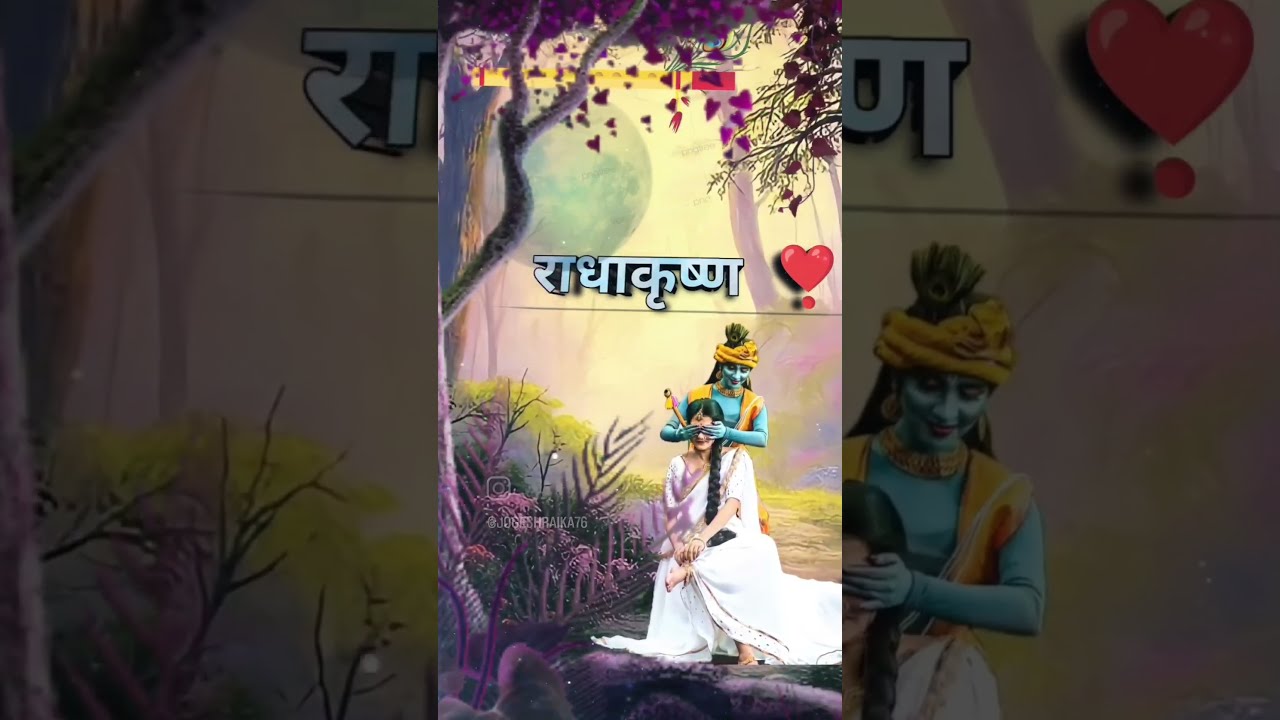In this vibrant, fantasy-themed graphic design image, two women are depicted in a mesmerizing forest setting. One woman, seated and wearing a long white gown with a black braid cascading over her shoulder, has her eyes gently covered by the hands of a second woman standing behind her. This second woman has striking blue skin and is adorned with a yellow turban-like wrap around her head and a matching yellow top. She stands out with a warm smile as she playfully engages with the seated woman. Surrounding them is a richly detailed landscape featuring green grass, purple trees, various plants, and dirt trails. Above them, tree branches and falling heart-shaped petals add to the enchanting atmosphere. In the distance, a close, greenish-gray moon looms large against the sky. Additionally, blue lettering in Arabic script stretches across the middle of the image, while a red heart is visible on the right side, enhancing the whimsical charm of the scene.